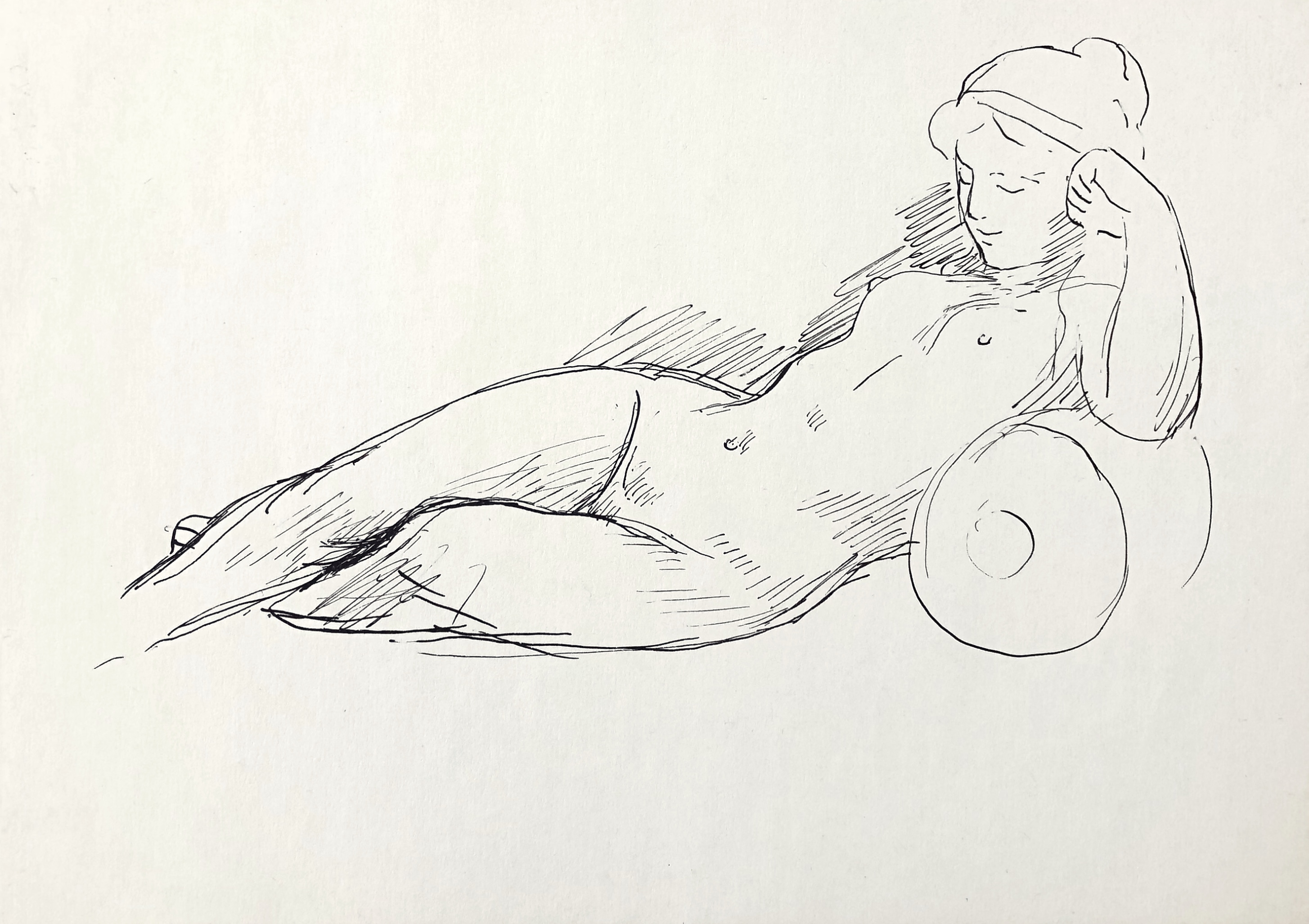The sketch is a simplistic, black-and-white drawing of a nude woman reclining on her left side, created using either pencil or pen on white paper. The woman is smiling subtly with her eyes closed, her head propped up and resting against her left hand, which is formed into a fist. Her left elbow is supported by a cylindrical cushion that adds depth and texture to the drawing. Her hair is parted in the center, pulled back into a bun, and secured with a headband. The sketch, which lacks the foot of her right leg, shows her left leg tucked under her right leg. The shading technique, achieved by moving the pencil back and forth, accentuates the shadows and adds texture, highlighting the contours of her body and the cushion. The image spans horizontally, capturing the woman in a relaxed, lounging position, with the cushion placed towards the right center of the composition.